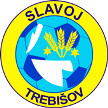The image depicts a circular insignia with a distinctive yellow outer border that is highlighted by blue strips on both the outer and inner edges. The top of the yellow area is inscribed with the Eastern European word "Slavoj," and the bottom with "Trebizov," suggesting it is affiliated with a football club. Centrally, the insignia features a stylized soccer ball comprising light and dark blue panels. Flanking the soccer ball are artistic depictions of golden wheat and white elements resembling knives from a plow, or blades, indicative of possible agricultural symbolism. The golden wheat is accompanied by stars, enhancing the design's intricate detailing. This patch-like insignia with its vivid imagery and lettering likely represents the Slavoj Trebizov football club.